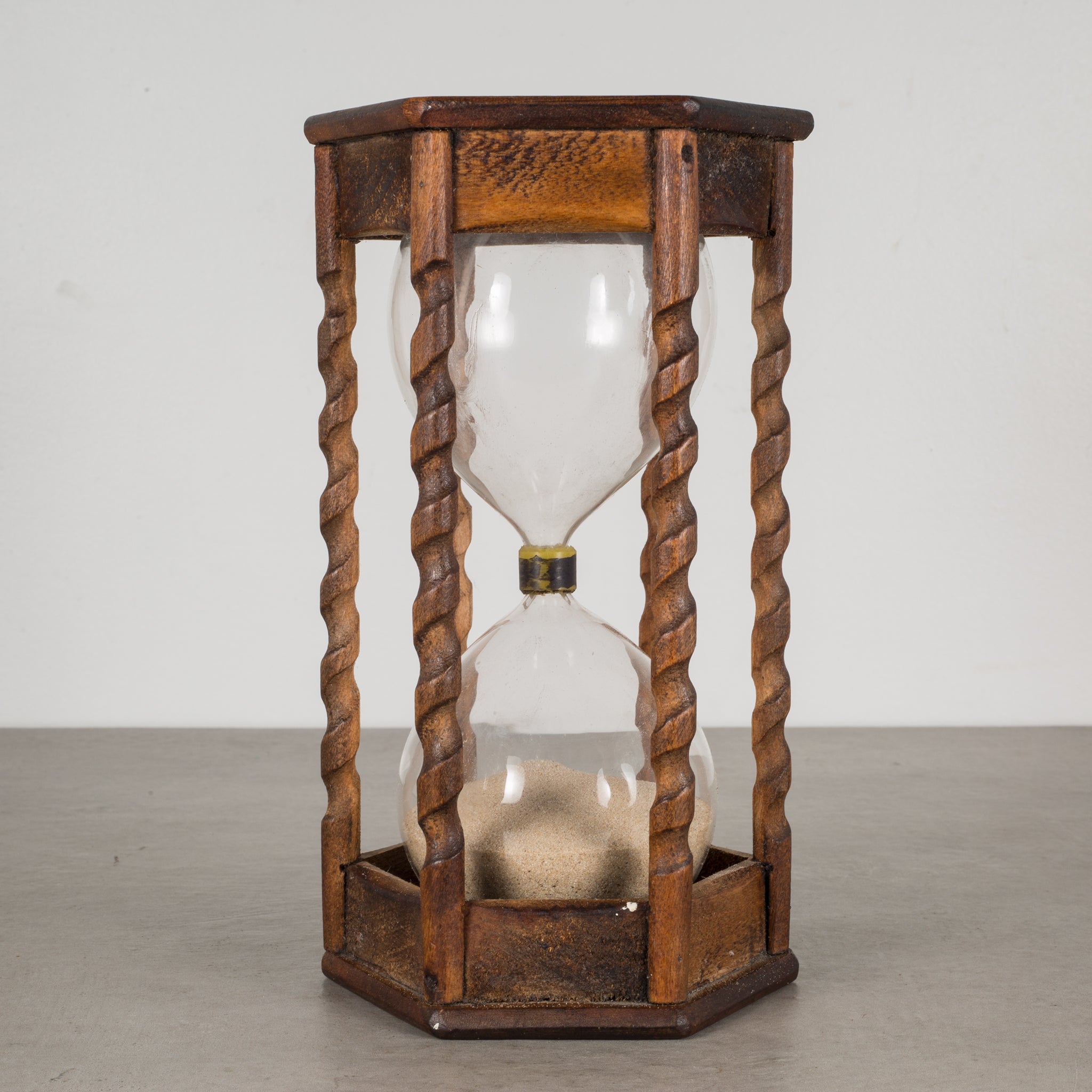The photograph, taken indoors against a pale grey, almost white wall, features a striking, hand-carved wooden hourglass sitting centrally on a light grey surface. The hourglass itself is encased in a hexagonal wooden stand consisting of intricately designed, spiraling columns that support the top and bottom wooden discs. These six columns showcase expert craftsmanship with their delicate twists and turns. The wood has a rich contrast in coloration; the top disc appears more orange with dark brown accents, while the bottom maintains a consistent darker brown hue. 

The hourglass is made of clear glass, through which you can see fine, light brown sand that has all settled at the bottom, filling approximately one-fourth to one-fifth of the lower chamber. In the middle of the glass, there is a distinctive yellow ring with a dark strip encircling it, which adds a unique focal point to the sand timer. The overall design combines a rustic elegance with functional artistry, inviting admiration and curiosity as it sits poised for its next turn.